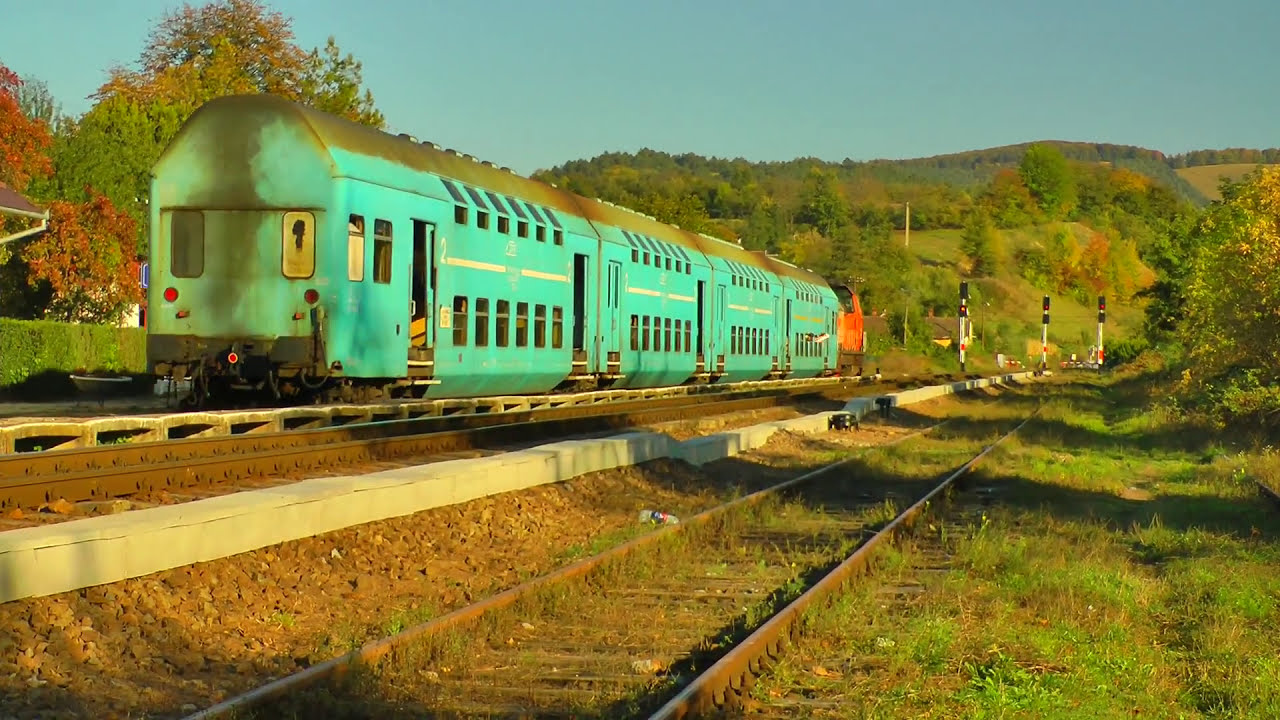The image is a detailed, color photograph taken in landscape orientation. It showcases a vintage train with four light aqua-colored cars and a red caboose on the leftmost set of tracks. Each car features distinct sets of doors, with varying states—some open, some closed. The train, appearing worn and slightly rusted, is positioned on the tracks which are surrounded by green grass. Adjacent to these tracks on the right are empty tracks, separated by a white concrete barrier. Further to the right lies another track running down the center, leading towards the horizon. At the end of the tracks, there are three sets of lights with red and yellow bulbs. In the background, rolling hills with trees shedding amber leaves are visible under a clear blue sky. Near the end of the tracks, an orange and red blotch resembling a fire adds a dramatic element. The overall perspective of the photo gives depth, with the train diminishing in size as it recedes into the distance.